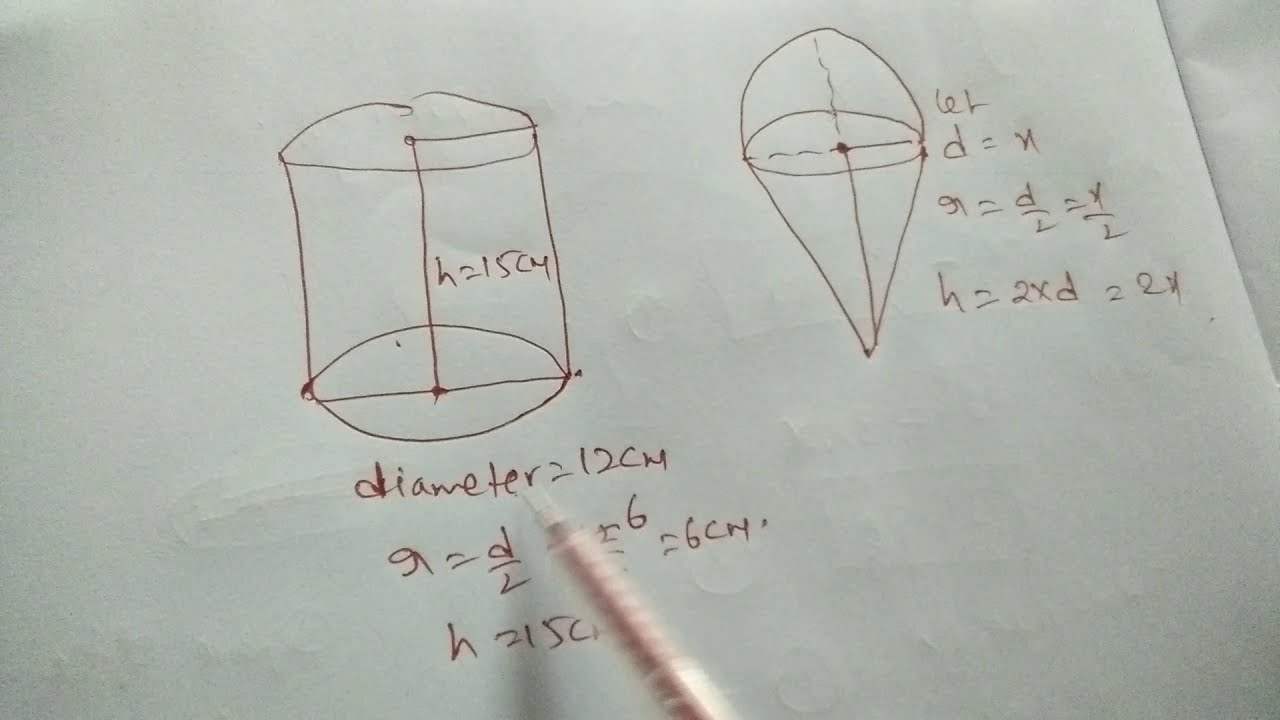The image is a photograph of a slightly wrinkled piece of white paper filled with geometric diagrams and mathematical formulas, drawn in pencil. On the left side, there is a detailed 3D drawing of a cylinder labeled "H = 15 centimeters" with the diameter noted as "diameter = 12 centimeters." The cylinder also includes a formula "D divided by 2 possibly equals 6 centimeters." Moving to the bottom of the cylinder drawing, the formula reads "H = 15 centimeters."

On the right side, there is a 3D cone with a smaller shape reminiscent of an ice cream cone on top. This cone is annotated with "6L," and below that, "D = N" followed by the equation, "π = D/L = Y/L." Further below, it specifies "H = 2X" and "D = 2X." The paper also shows some additional shapes and symbols that are not entirely legible, leading into more equations involving terms like "2 times." In the foreground, a blurry pen or pencil is visible, indicating movement during the picture taking, adding to the sketchy and detailed nature of the document. Indentations from something written on the reverse side of the paper are also faintly visible, contributing to the overall texture and complexity of the image.